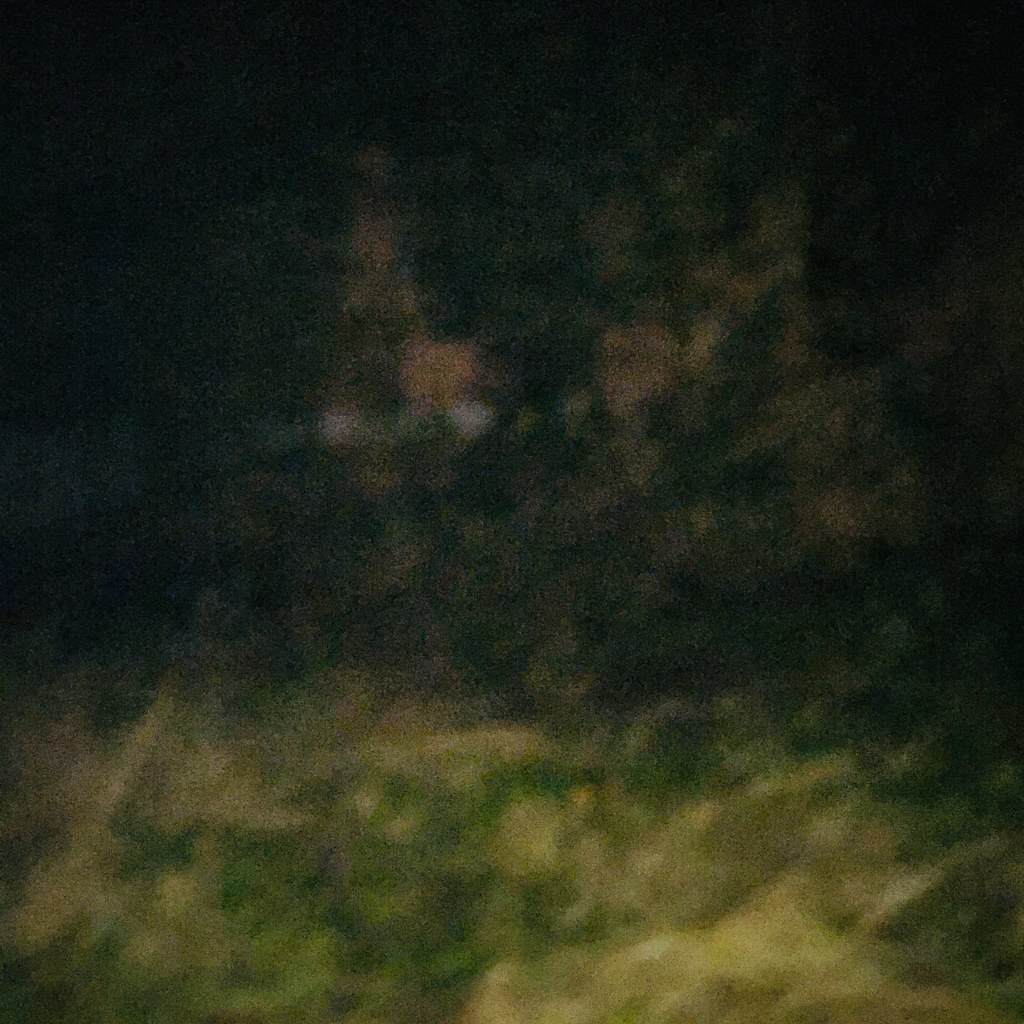This image, which appears to have been taken at night, is extremely blurry and dark. The upper portion is almost completely black, indicating nighttime, with some very dark coloring around the edges. The bottom third of the image features a mix of greens, beiges, and browns, suggesting patches of grass that might not be entirely healthy, potentially interspersed with dirt or straw-like lines. The right-hand side shows more olive green and brown, while the back and left sides are a mix of green and beige, possibly indicating tree branches or leaves changing color. Scattered throughout the image are white dots that could be specular reflections or artifacts from the photograph itself. Despite the visible elements, the blurriness and darkness make it difficult to definitively interpret the exact contents of the photo, and there are no clear signs of people, animals, plants, buildings, or any other objects.